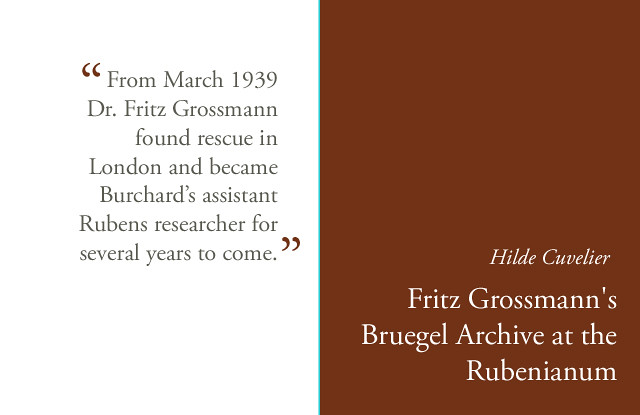The image features a predominantly white background. On the left side, there's a gray quotation that reads, "From March 1939, Dr. Fritz Grossman found rescue in London and became Burchard's assistant, Rubens researcher for several years to come." This text is presented in a light gray font, with the quotation marks matching the brown color of the rectangle on the right. On the right side of the image is a brown rectangle, longer in height than width. At the bottom of this rectangle, the words "Hilde Cuvelier, Fritz Grossman's Bruegel archive at the Rubinianum" are printed in white text. The content appears to be part of an exhibit or informational sheet, with no other objects or people in the image.